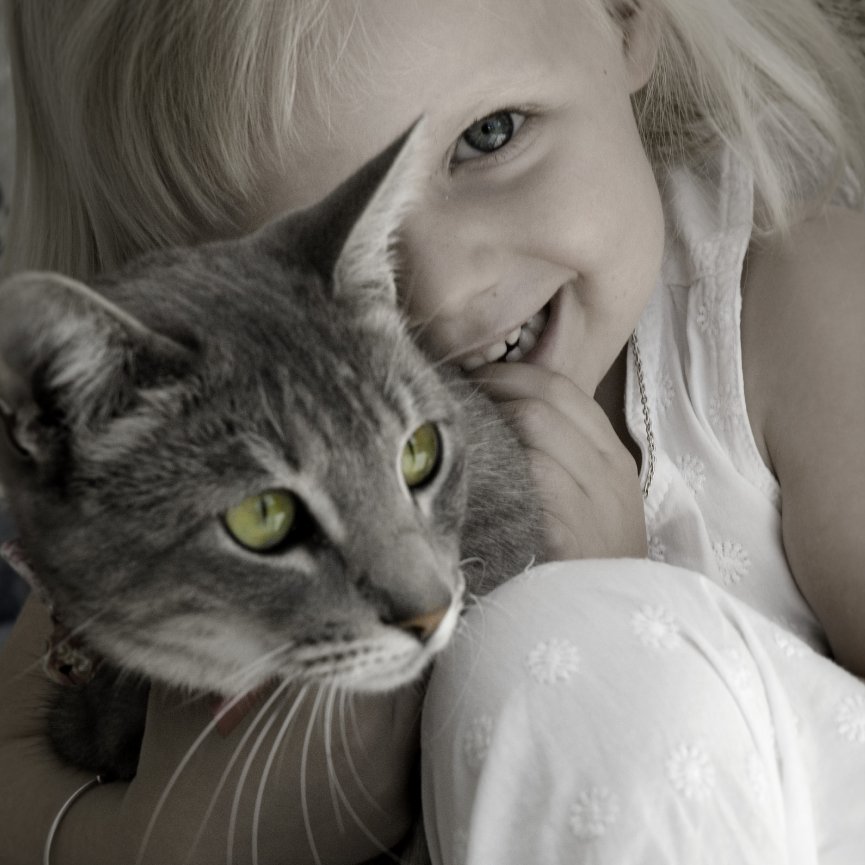This photograph features a smiling little girl with blonde hair, dressed in a white outfit adorned with small daisy flowers. She is positioned near the center of the frame, emerging from the upper right corner. Her left hand rests on her lower lip, and she is affectionately holding a gray cat with green eyes. The cat, nestled in the girl's arms, obscures her right eye and part of her mouth and nose, while its white whiskers stand out prominently. The cat gazes to the right side of the photograph, aligning with the girl's left. The composition emphasizes soft, light tones, focusing on the interplay between the girl's bright attire and the cat's gray fur. No markings or photographer's name are visible, suggesting an art photography style rather than a personal snapshot.